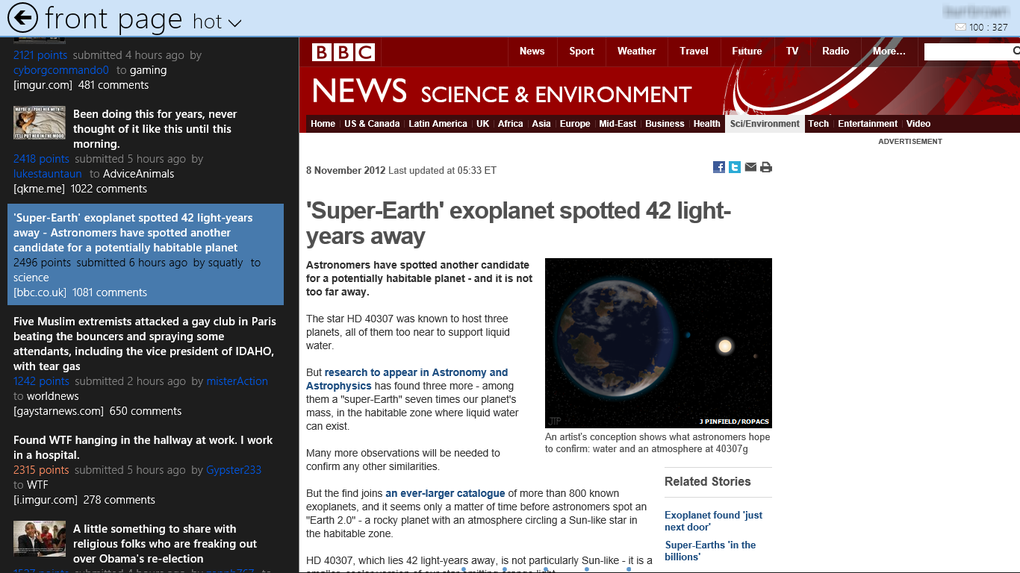The image depicts a webpage viewed on a laptop or desktop computer. The top of the page features a light blue banner. On the left side of the banner, there's a circle with a black arrow pointing to the left, accompanied by the text "front page" in lowercase letters and "hot" followed by an inverted triangle without its bottom. To the right, a battery symbol reads "100;327."

The left column is dense with content. At the top, it shows "2121 points submitted four hours ago by CyborgCommando2Gaming," with the text in shades of blue, gray, and white. Below that, there's a picture of a man and woman in bed with the caption, "Been doing this for years, never thought of it like this until this morning." This post lists "2418 points in blue, submitted five hours ago by Luke Staunton (in blue), two in gray, Advice Animals." Below, a link reads "QKMe.me" followed by "1022 comments" in white text.

Further down, a blue square reports, "Super Earth Expo: Planet spotted 42 light years away. Astronomers have spotted another candidate for a potentially habitable planet," in white lettering. This post has "2496 points, submitted six hours ago by Squatly2" in navy text, followed by "Science" in white, and "BBC.co.uk" in square parentheses and "1081 comments."

Beneath, text reads, "Five Muslim extremists attacked a gay club in Paris, beating the bouncers and spraying some attendees, including the vice president of Idaho, with tear gas." Below, there are additional listings and a blurry photo.

The right column starts with a red banner at the top displaying "BBC News, Sports, Weather, Travel, Future TV, Radio, More," followed by categories such as "News," "Science and Environment," and a black banner with "Home" and a list of continents, "Business, Health, Tech, Entertainment, Video."

An article with a white background and titled "Super Earth Expo: Planet spotted 42 light years away," spans three to four paragraphs. At the bottom of the article, "Related Stories" lists two more stories in blue text.